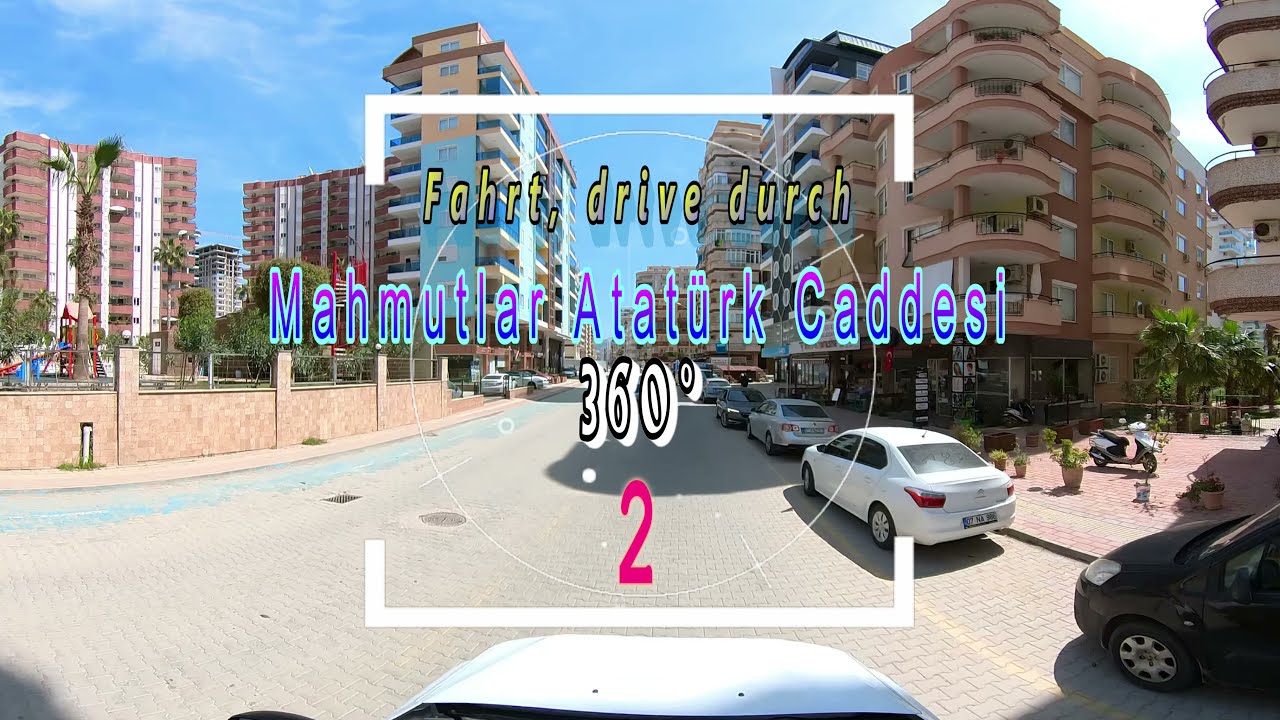The image depicts a modern street scene lined with tall apartment buildings, most of which feature balconies. The street, composed of black and light gray cobblestones, runs down the middle with parked cars and a motorcycle positioned on the right-hand side. Some palm trees and various plants are visible along the sides, with a small playground and additional trees on the left-hand side. Central to the image is a white-outlined square, partially open on the left and right sides. This square contains a layered text description: in yellow letters, "FAHRT, drive DURCH" appears at the top; beneath it, the phrase "Mamluktar Atatürk Caddesi" is written in a blue and purple gradient; followed by "360 degrees" in white letters framed in black, and a pink number "2" at the bottom. The street is mostly empty of people, emphasizing the architecture and the distinct textual overlay.